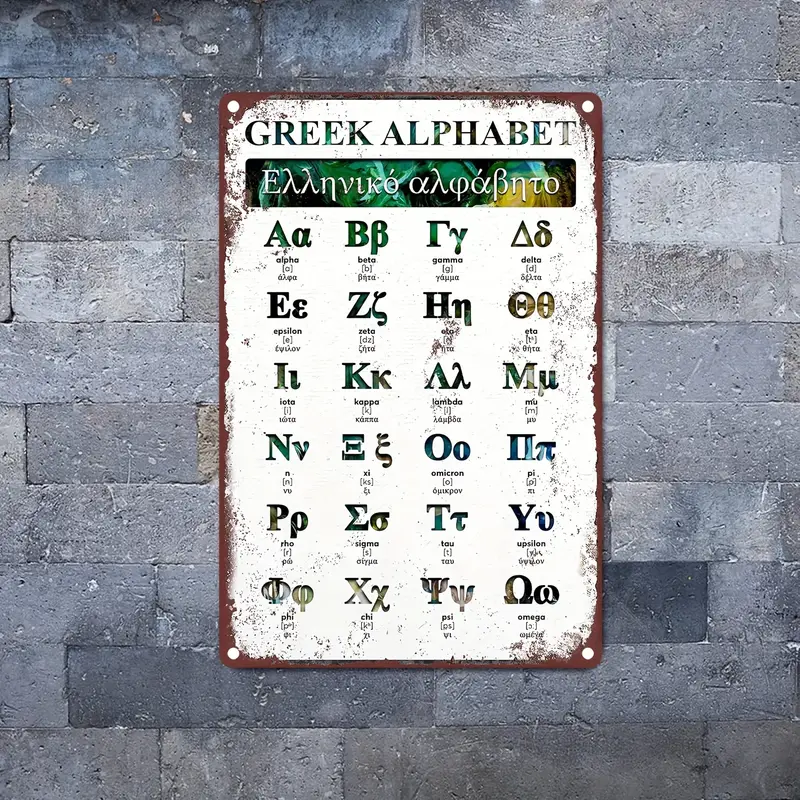The image presents an infographic of the Greek alphabet displayed on what appears to be an old-fashioned, tin-like metal sign with rivets in each corner, giving it a vintage or weathered look. This sign, trimmed in red, prominently features the Greek alphabet in the center. Along the top, the title "Greek Alphabet" is written, followed by a rectangular green section with text in Greek that is difficult to read. The alphabet itself consists of all 24 Greek letters, neatly organized into six columns of four rows each. Each letter is shown in both uppercase and lowercase, with its corresponding English name underneath. The background of the image is a gray brick wall, giving the impression of an aged and textured backdrop, potentially enhancing the historic aesthetic of the overall composition.